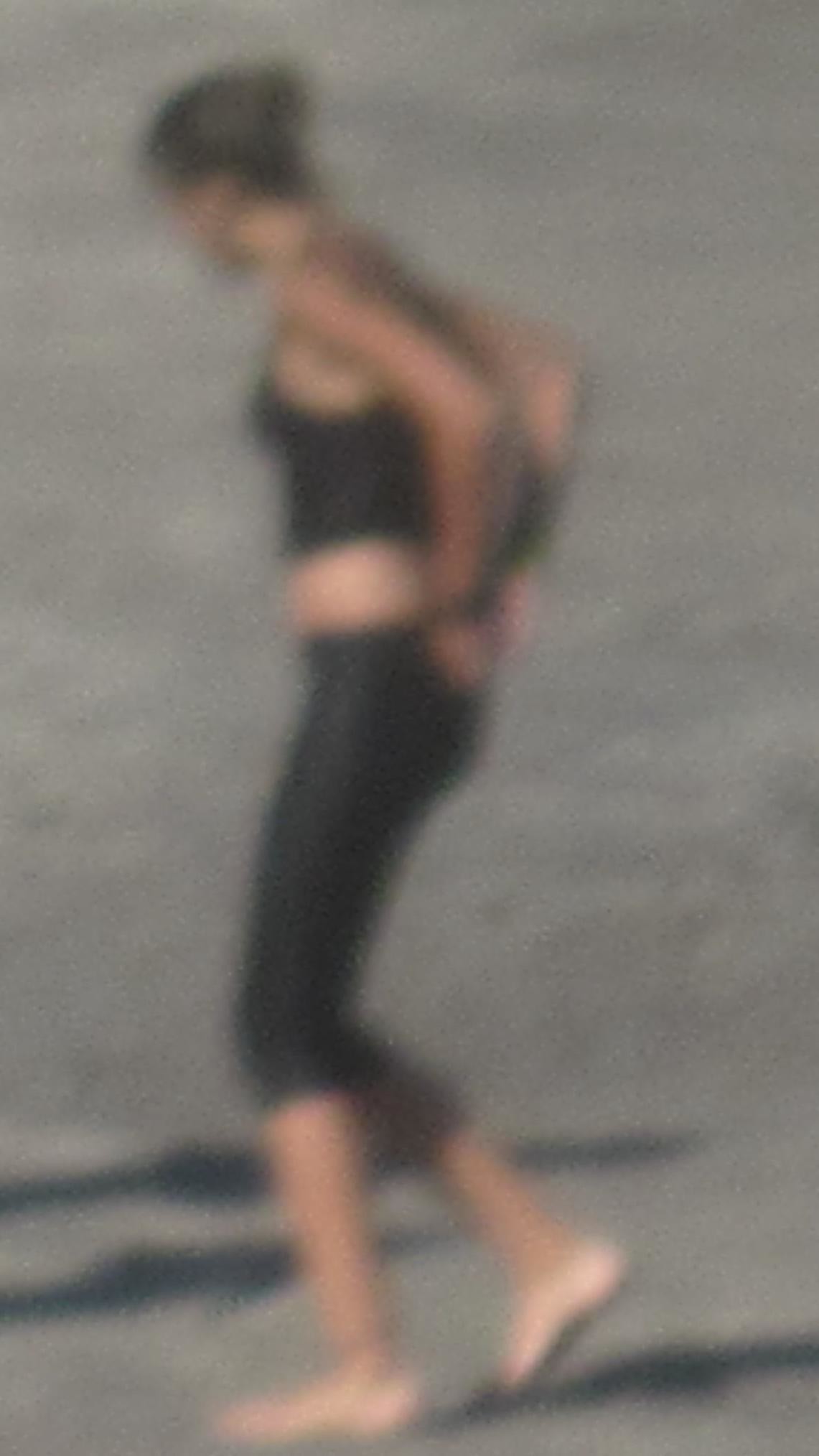This photograph, though slightly out of focus, captures a moment of an athletic woman walking on concrete. She is barefoot, suggesting she may have just finished a run or some sporting activity. Her brown hair is neatly tied into a bun at the back of her head. She wears a black tank top paired with Capri-length workout pants or a leotard, accentuating her fit physique. The woman’s arms are positioned behind her, hands resting on the back waistband of her pants. A wristwatch is visible on her left wrist, though the blur makes it hard to determine its exact model. The scene conveys a sense of completion and possibly exhaustion, as if she has just crossed the finish line of a race or concluded an intense workout session.